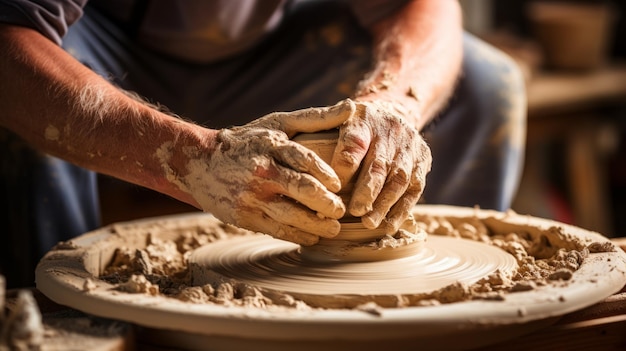In this detailed image, we see a potter deeply engrossed in shaping a piece of clay on a rotating pottery wheel. The potter's clay-covered hands are prominently visible, emerging from the top and middle left of the image, working meticulously to mold the wet clay directly in the center of the shot. The skilled hands are bare and coated with thick layers of clay. The potter's attire includes a greenish-gray shirt with sleeves rolled up and blue trousers, both stained with mud. He is seated, most likely on a stool, and focused intently on his craft in broad daylight, as sunlight illuminates his hands and surrounding objects. The workspace is somewhat cluttered with clumps of clay scattered around the wheel, adding to the scene's authenticity. In the blurred background, on the right side of the image, there are several brown-colored pottery items, indicative of the potter's previous works, adding depth and context to the photograph.